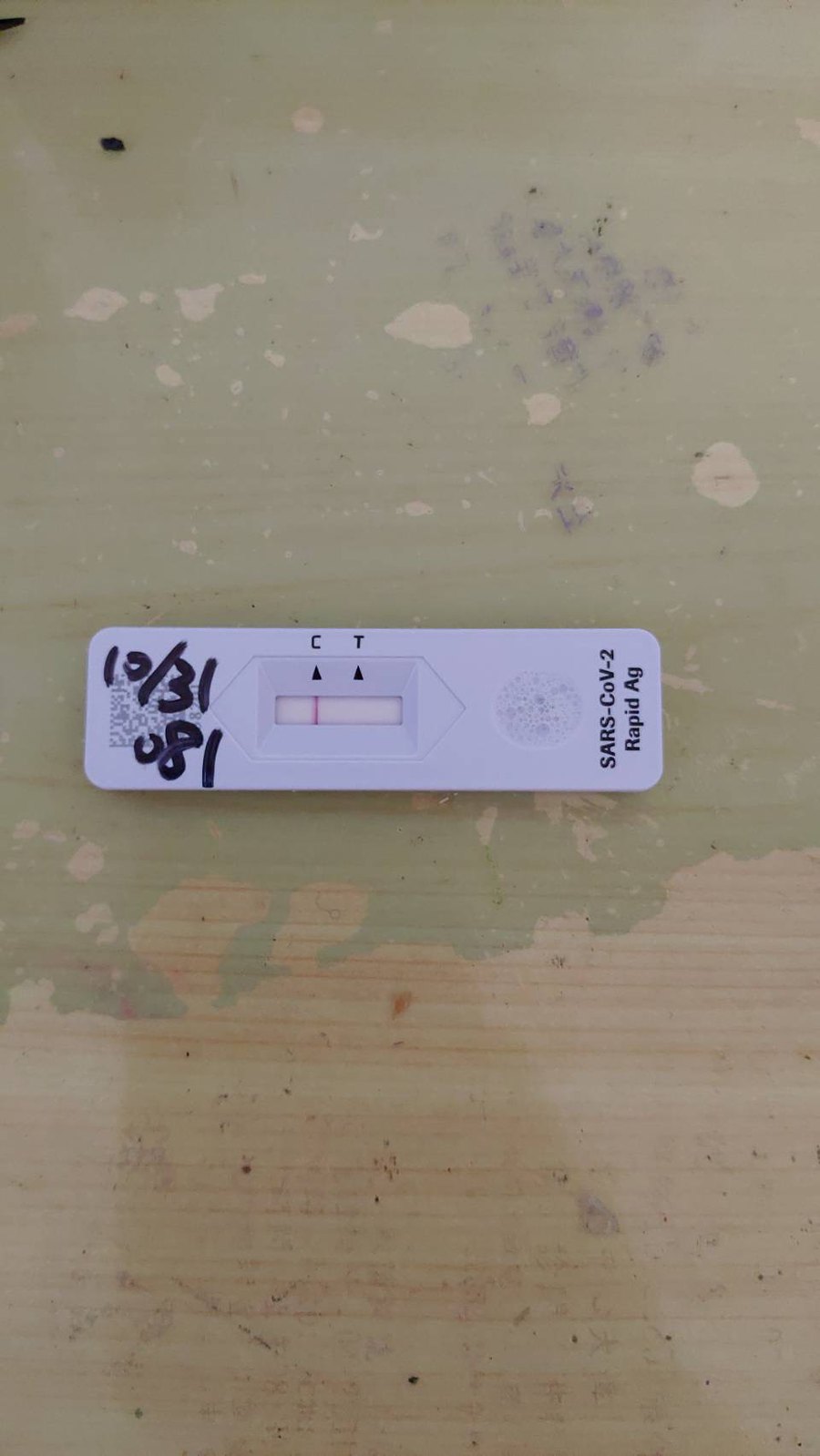On a light-colored wooden table with a faded, light green top, a COVID-19 rapid antigen test is prominently placed horizontally in the center. The table's green paint appears to have worn off and dripped in some areas. The COVID test features a label in black font on the bottom right that reads “SARS-CoV-2 Rapid Ag.” On the left side of the test, the date "10-31" is handwritten in marker, with a partially legible secondary marking that might read "081" or "18" upside down. The test’s result window, a small white rectangle in the middle, displays a single red line beneath a black triangle pointing to a "C," indicating a negative test result. Another black triangle points to a "T," which remains unmarked, further confirming the negative status of the test.